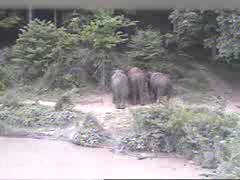The photograph is a small, possibly old or filtered color image that appears faded and difficult to discern. At the center of the image are three roundish, oblong objects which, upon closer inspection, seem to be elephants viewed from behind, although discerning their details, such as trunks or tusks, is challenging. The foreground is almost white and could be sand or water, with some greyed-out but detectable vegetation. The area surrounding the elephants also appears white. Behind them, there is denser, darker vegetation resembling a jungle or forest, with taller trees. The top of the image features a curious grey line, and there is a thin black line at the bottom right that blends into the vegetation. A small structure or building is vaguely visible in the background amongst the trees. The overall perspective and distance make the subjects difficult to distinguish clearly, contributing to an impression of movement or blur, making it hard to confirm the exact scene.